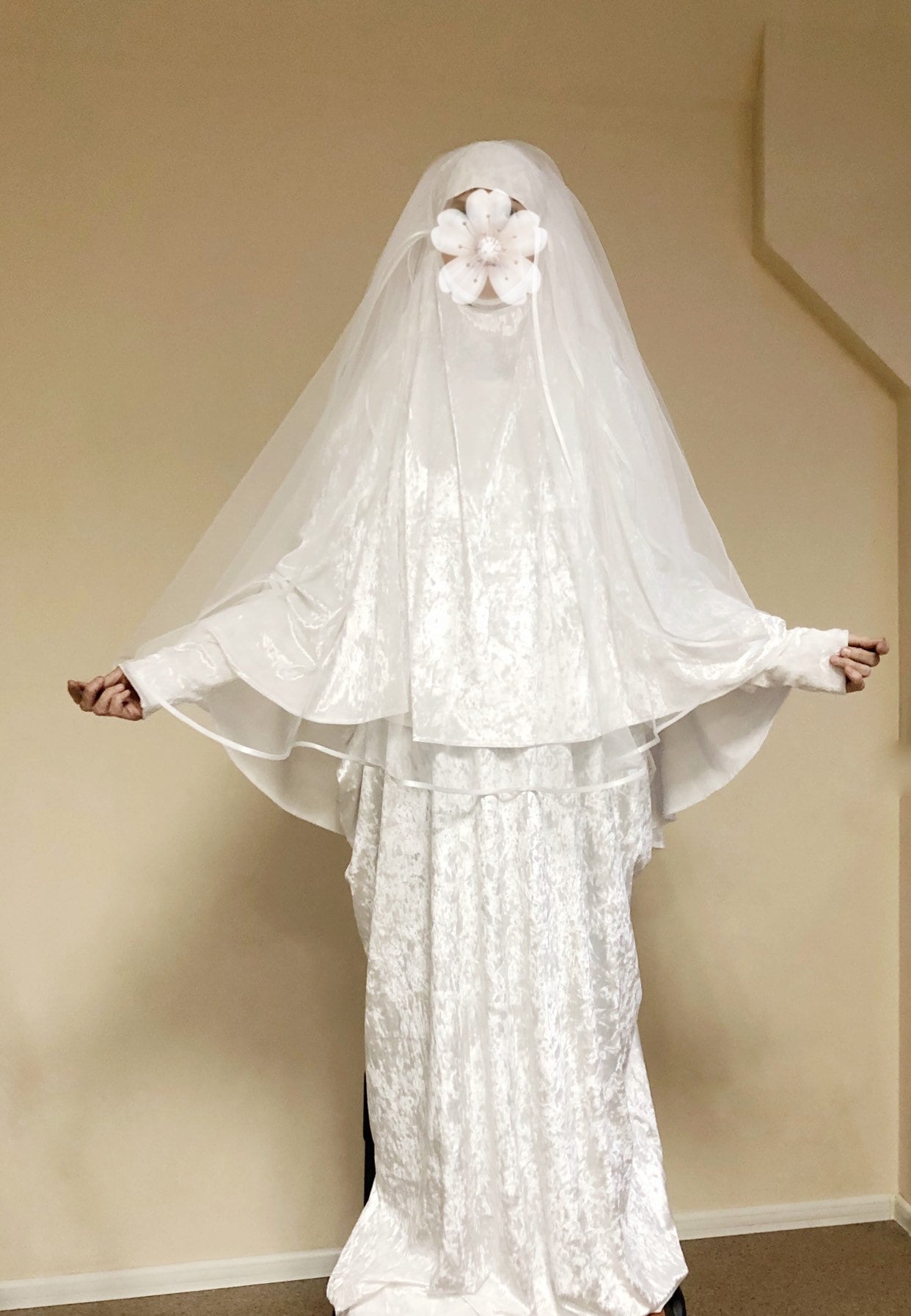In the photo, a woman stands in a meticulously embroidered white dress that reaches down to the floor, adorned with floral designs. The long sleeves extend past her palms, ending at her fingertips as she holds the dress out to her sides. Her arms are slightly outstretched, showcasing the elegance of the gown. She wears a translucent white veil that cascades down below her waist, and her face is notably obscured by a fully open white flower, adding an intriguing element of anonymity to her appearance. Behind her, a light brown wall provides a neutral background, with a distinctive protrusion in the top right corner creating an unusual angular shape. The floor is covered with a dark brown carpet, adding contrast to the scene. The setting and attire suggest that she might be a bride, possibly preparing for her wedding ceremony.